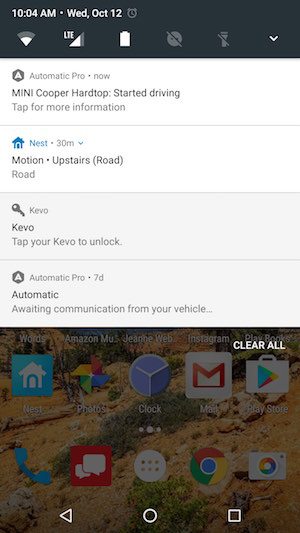The image is a screen capture from a smartphone, displaying the phone's status bar and notifications. At the very top, in small letters, the time is shown as 10:04 a.m. on Wednesday, October 12th. Adjacent to the time and date are several status icons: a Wi-Fi icon, an LTE 4G connection icon, a fully charged battery icon, an icon with a diagonal line indicating a disabled feature, another icon showing a disabled flashlight, and a pull-down arrow.

Below the status bar, a series of notifications are displayed within rectangular sections. The first bar reads: "Automatic Pro: Mini Cooper Hardtop started driving. Tap for more information." The second bar displays a notification from Nest: "Motion detected Upstairs 30 minutes ago." The third bar is from Kivo: “Kivo: Tap your Kivo to unlock.” The fourth bar is another notification from Automatic Pro stating: "Awaiting Communication from Your Vehicle."

At the bottom of the screen, a row of app icons is visible, including Home, Google Photos, Clock, Gmail, Play Store, Phone, Messages, App Drawer (six dots in a circle), Google Chrome, Camera, and a shopping-related icon. Finally, the navigation bar at the bottom shows the Back button, the Home button, and the Square button for switching between programs.